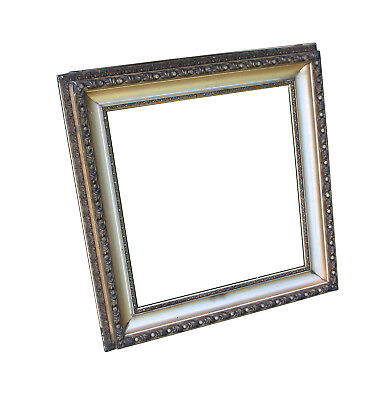The image depicts an ornate, square picture frame photographed at an angle, creating a slightly skewed perspective where the top and left sides appear larger than the right and bottom. The frame is primarily metallic silver or perhaps wooden with a golden finish, adorned with intricate filigree and relief patterns that enhance its detailed texture. The central portion of the frame is a flat white matte that matches the plain white background, giving the frame a floating appearance. The image is devoid of any content within the frame or any discernible background, suggesting it could be a product photo intended for a website, showcasing just the frame itself with no text or additional elements.